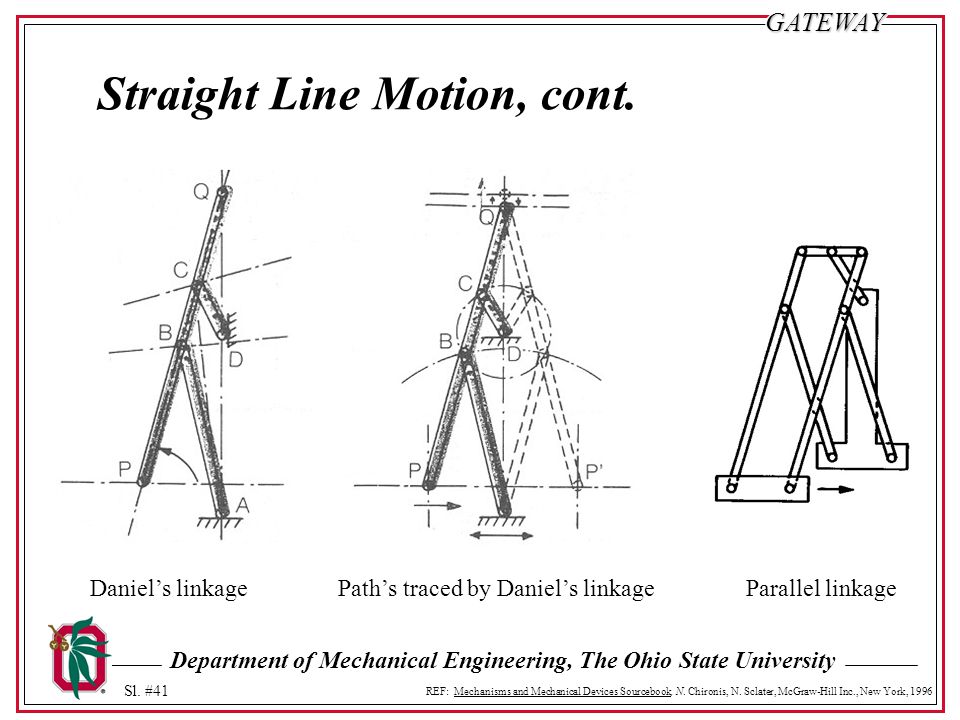This image is an informational page with a white background, bordered by a red outline and a thin black interior border adjacent to the red one. In the upper right-hand corner, the word "GATEWAY" appears in all caps and black letters. The left-aligned title in bold black letters reads, "Straight Line Motion, C-O-N-T."

Centered on the page are three diagrams featuring various lines and letters, such as Q, C, B, D, P, and A. The first diagram on the left and the middle diagram display a horizontal line and an upside-down V shape that forms a triangle at its peak. The third diagram on the right resembles the outline of connected bars. Underneath the left diagram, the caption reads "Daniel's Linkage," beneath the middle diagram it says "Paths Traced by Daniel's Linkage," and under the rightmost diagram, it reads "Parallel Linkage."

At the bottom of the page, centered within the border, the text "Department of Mechanical Engineering, The Ohio State University" is displayed. Additionally, there is a logo located at the bottom left featuring a red-bordered square with green leaves inside. The primary color scheme of the image is black, white, and gray, with red and green accents, and the overall style suggests it is part of an educational presentation or book related to engineering.